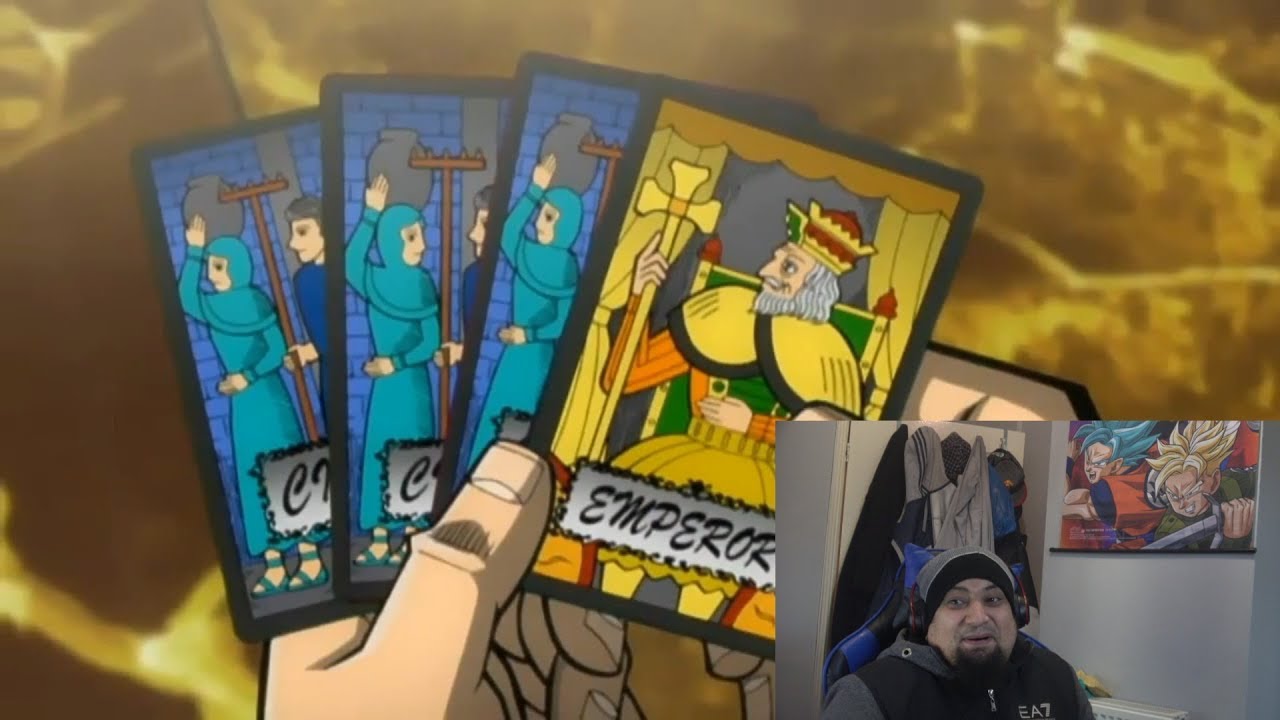The image is a detailed composite, primarily featuring a cartoon-style illustration with an inset photograph of a man in the bottom right. The cartoon depicts a pair of hands holding four cards, three of which are blue and identical, showing a woman with a water jug on her head and a man with a rake beside her, set against a golden floor background. The fourth card stands out with a golden yellow color and is labeled "Emperor," depicting a king on a throne.

In the inset photograph, a man is seen wearing a hoodie and headphones, looking amusedly at the screen. Behind him, the wall features hanging clothes and a poster of an anime character, indicating his interest in animation. The photograph overlaps slightly with the cartoon, covering part of the right hand. The scene likely captures the man creating a reaction or instructional video about the animated card game he is observing, possibly for a platform like YouTube or TikTok.